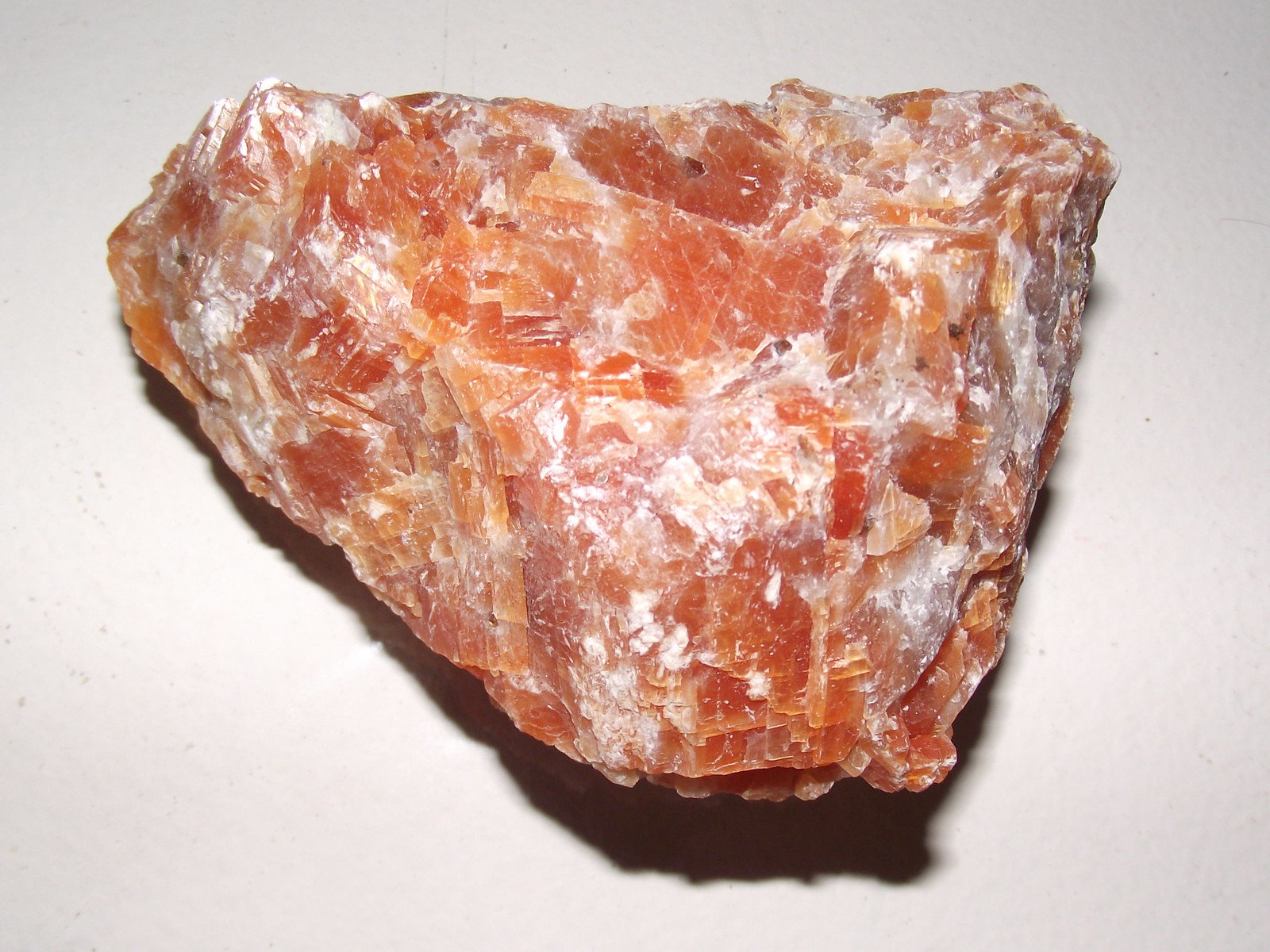This photograph captures an intriguing and unique rock formation, resembling a crystallized stone, showcasing an inverted triangular shape with broken-off points. The rock is characterized by alternating bands of burnt orange and opaque white crystals, enhancing its striking appearance. Its surface is flat with some concave areas, and the sides appear chiselled into flat planes. The rock is set against a white, light grayish-blue background, casting a shadow from the top left corner to the bottom right. The absence of reference objects makes it challenging to determine its exact size, which could range from a small fragment to a larger formation. Evoking a sense of geological history, the rock seems to have been formed over eons, potentially in a cave, through the gradual deposition of minerals by flowing water.